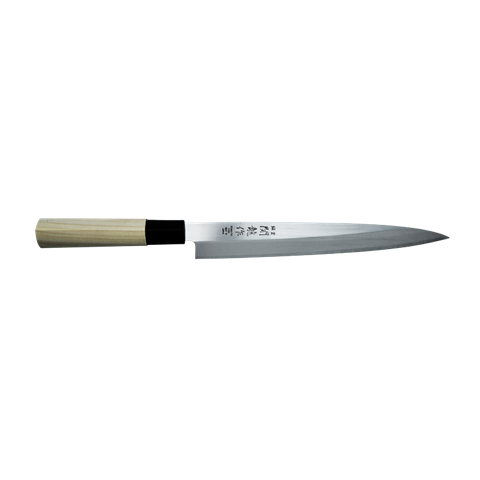This image showcases an elegant, high-end knife that appears to be of Japanese or Chinese origin, implied by the intricate characters etched on the blade. The text, however, is unreadable. The knife is presented against a pure white background, making it appear to float. Its handle, constructed from a light brown or pale beige wood, is cylindrical and about 3 inches long. A black piece, blending with the handle, secures the blade. The blade itself is silver, flat, and extremely sharp, tapering to a fine point with a line down its center indicating two different thicknesses. It resembles a fillet or sashimi knife, though it shares qualities with a butcher knife, measuring approximately 7 to 8 inches in length. The lack of serrations on the blade reinforces its professional and refined design.